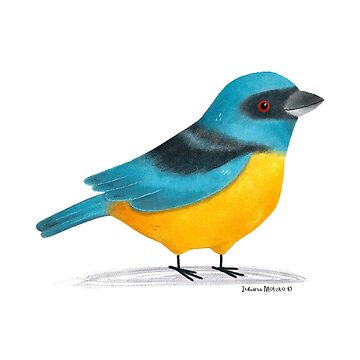This painted, animated image features a vividly colored bird standing on a simple white background. The bird, depicted in a possible watercolor style, showcases a dominant blue hue on its head, back, wings, and tail. It has a striking yellow chest and stomach, and a distinguished black band encircles its beak and eye area, with another black band over the crest of its wing. The bird is detailed with a short, broad beak reminiscent of a finch and possesses a reddish eye that adds a pop of contrast to its color palette. The bird’s black feet are simplistically drawn and lack realistic detailing, standing atop a gray, scribbled shadow. Below this shadow lies the artist’s signature, which is too small to decipher. Predominant colors in this illustration include blue, black, yellow, white, and a small red accent in the eye. Despite the simplistic background, the bird stands out vividly with its colorful and abstract design elements.